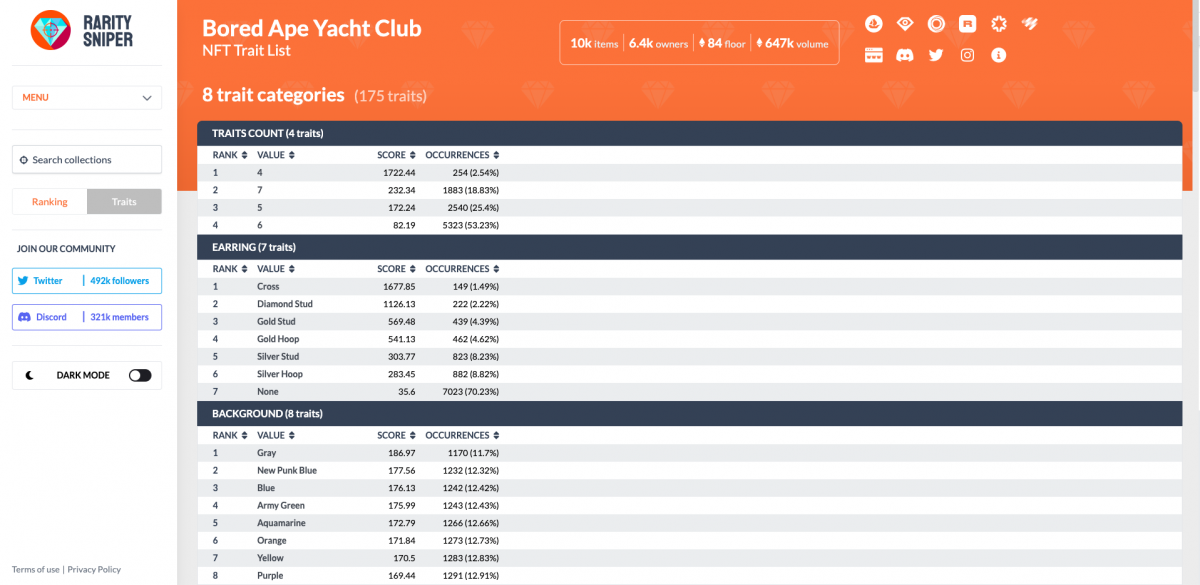The screenshot captures a section of a website titled "Rarity Sniper," marked by a small icon featuring blue, red, and orange colors on the left. Dominating the page is a large rectangular orange box containing key information about the "Bored Ape Yacht Club NFT Trait List." The text within this box notes that there are 8 trait categories comprising a total of 175 traits. Additionally, it provides statistical data including 10,000 items, 6,400 owners, a floor price of 84, and a trading volume of 647k.

To the right of the main content are several white icons arrayed in two rows, with six icons on the top row and five on the bottom. These icons include recognizable ones such as Twitter and camera symbols.

Below the orange box, various trait categories and their details are listed. The first category is "Traits Count," followed by "Earring," and "Background." Each category includes specifics such as rankings, values, scores, and occurrences. 

On the left side of the page, a vertical menu features buttons including "Menu," "Search Collections," "Earring," "Traits," "Join Our Community," and quick access buttons for Twitter, Discord, and Dark Mode.